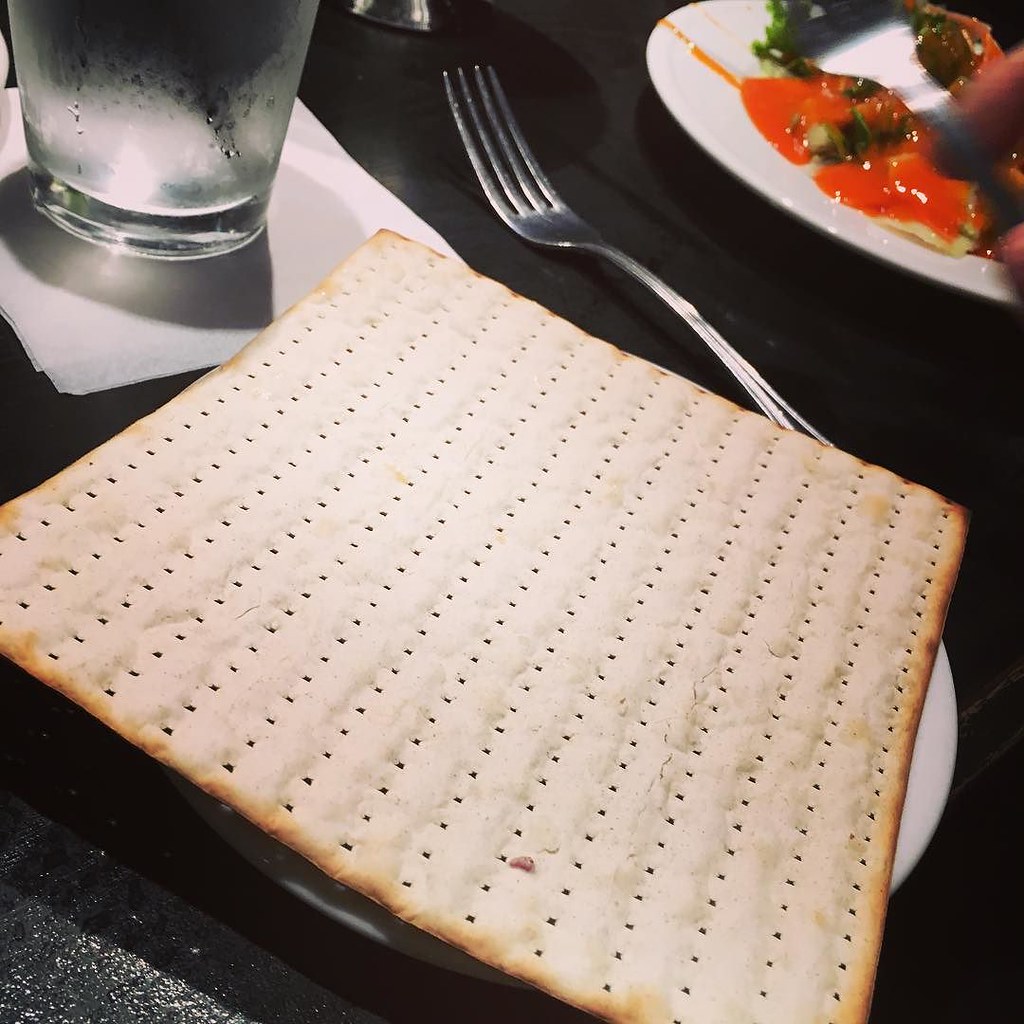This photograph features a close-up view of a table setting at a restaurant. Dominating the image is a large square piece of matzah bread with evenly spaced rows of punched holes and toasted brown edges, covering a white plate. The table is adorned with a black tablecloth, creating a striking contrast with the white dishware. To the left of the plate, there's a glass of water filled to the brim, resting on a white napkin with condensation visible on the outside of the glass. Above the matzah, there's another white plate that seems to hold a dish possibly consisting of pasta, likely ravioli, with a vibrant red sauce and some green vegetables. The edge of this secondary plate is smeared with red sauce, adding a casual touch. A fork is positioned to the far side of the main plate. The setting also hints at a human presence, with part of a thumb or finger visible near the edge of the frame, emphasizing the candid nature of the scene.